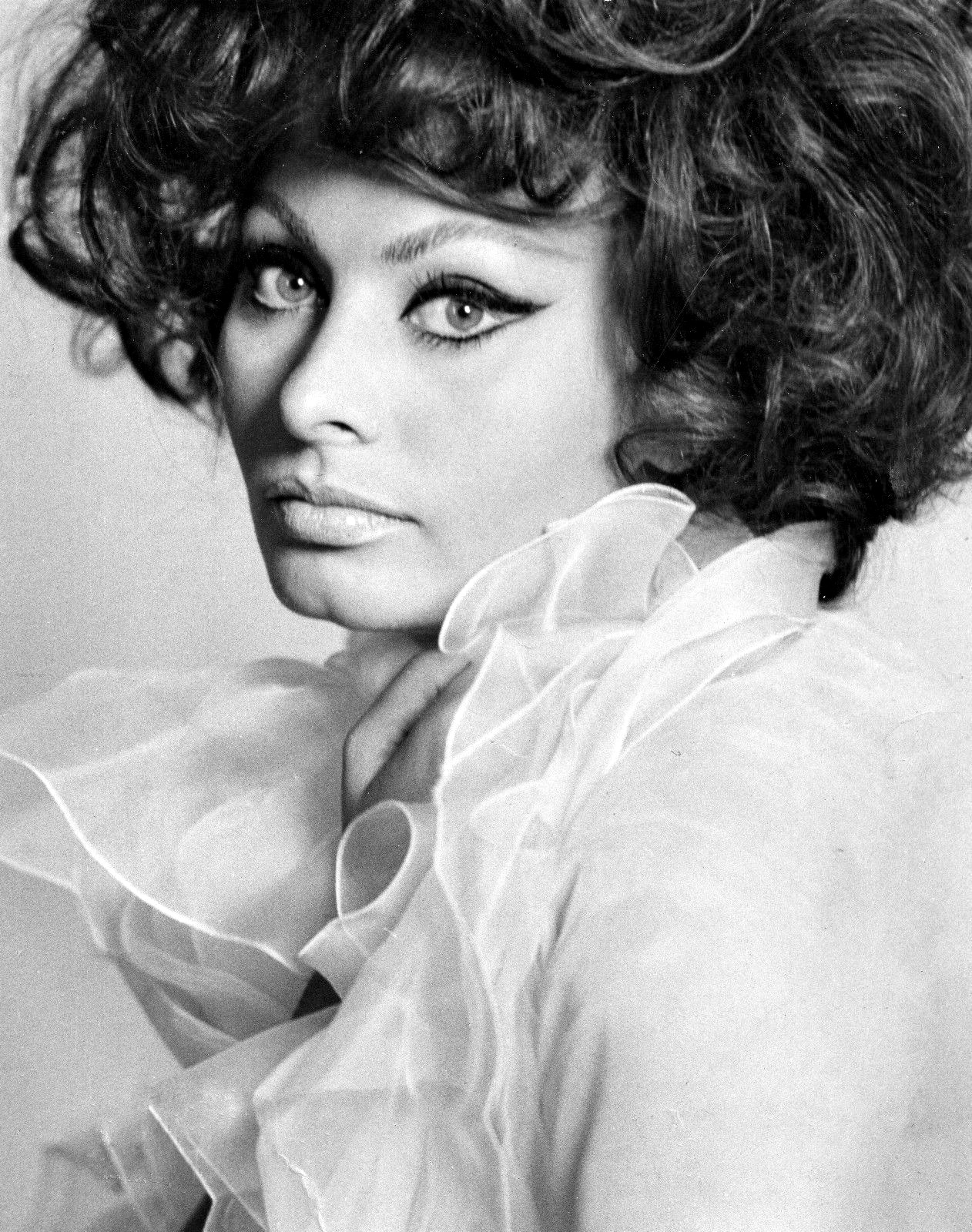This black-and-white publicity shot features the iconic Sophia Loren, her mesmerizing gaze fixed directly on the camera. The star's makeup showcases dramatic cat-eye eyeliner, accentuating her eyes with dark, winged lines that extend to a teardrop-like point at the corners. Loren is adorned in a delicate, semi-translucent white top, notable for its frilly collar that adds a touch of femininity and elegance to her look.

Her hairstyle is reminiscent of the voluminous styles of the 1960s and 70s, a voluminous arrangement that, while not quite a beehive, exudes a sophisticated, retro charm. The framing of the image cuts off part of her hair, placing additional emphasis on her captivating face. Her hand rests near her neck, partially obscured by her outfit, drawing further focus to her striking facial features. The image is devoid of any writing or additional elements, ensuring that all attention remains on Sophia Loren's timeless beauty.